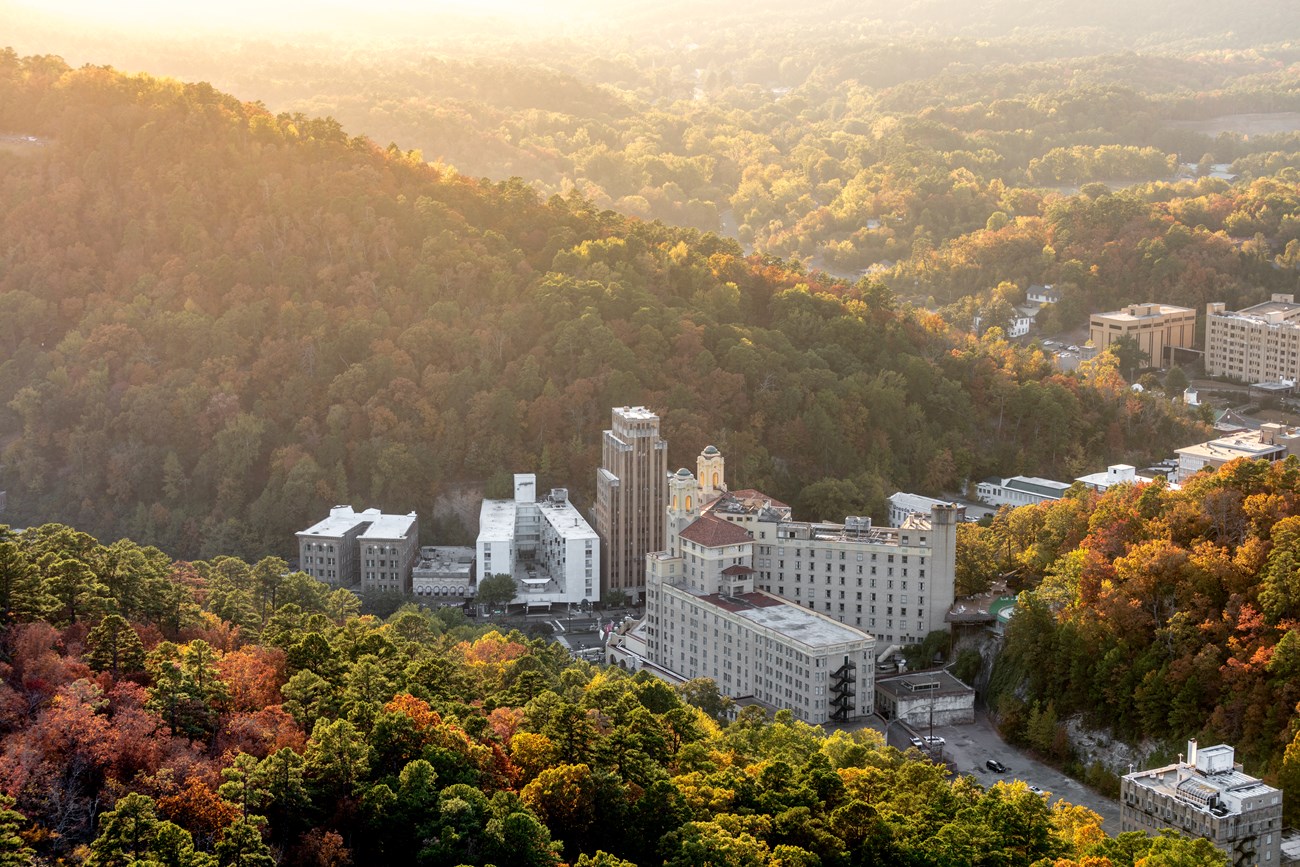This aerial photograph captures a sprawling city nestled within a valley bordered by rolling mountain ranges. On the left side of the image, a lush hillside is blanketed with green foliage, interspersed with the vibrant hues of autumn as leaves transition to red and orange. Central to the photo are several prominent high-rise buildings, some towering nearly to the scale of skyscrapers, displaying a historic architectural style. These buildings are likely hotels, characterized by distinctive features like blue domes and yellow, oval-shaped windows. Parking spaces and a few vehicles are visible, accentuating the urban setting. The serene beauty of the area is enhanced by the sunlight casting a pink and orange haze over the verdant landscape, creating a picturesque blend of natural and urban elements. On both the left and right sides of the central buildings, more trees exhibit a stunning mix of green with occasional bursts of red and yellow, adding to the overall tranquil and captivating scene.